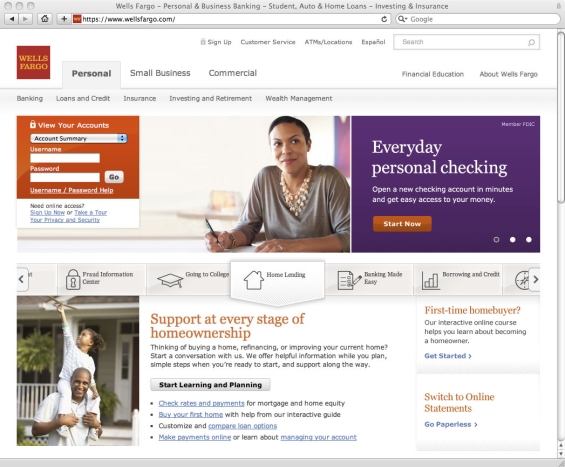The image displays the Wells Fargo homepage. The background of the webpage is predominantly white. At the very top, a grey toolbar features dark grey text on a lighter grey background, highlighting various categories such as "Wells Fargo," "Personal and Business Banking," "Student," "Auto and Home Loans," "Investing," and "Insurance." Beneath this toolbar, the address bar shows the URL "https://www.wellsfargo.com."

In the main section of the webpage, the Wells Fargo logo, consisting of yellow "Wells Fargo" text on a red square background, is prominently displayed. Below the logo, there is an image of a woman adorned with a three-strand gold necklace and wearing a grey long-sleeved top. She holds a black pen in her hand. To the right of the woman, a purple frame contains white text that reads, "Everyday Personal Banking."